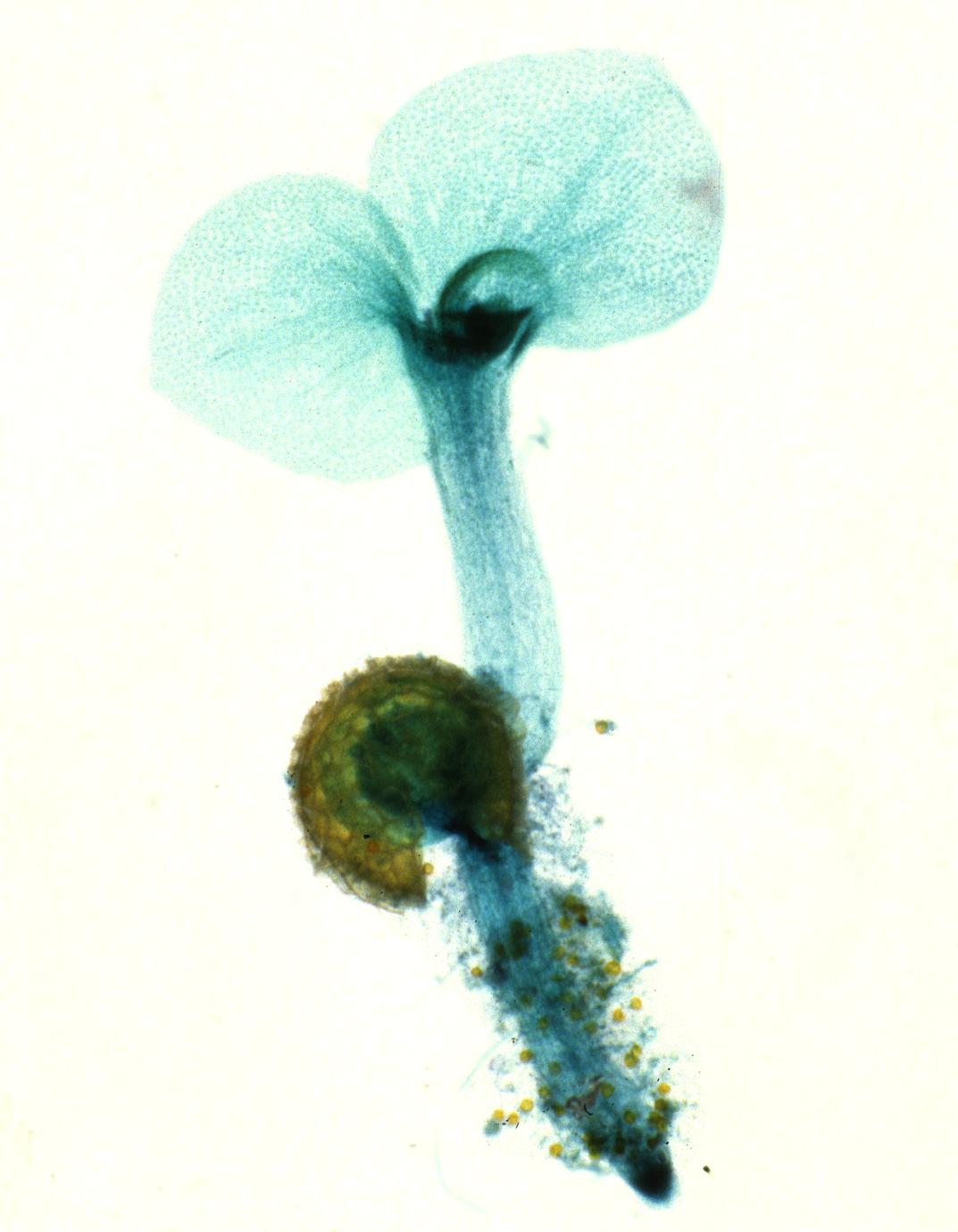The image depicts a botanical illustration or possibly a microscopic view of a plant cell, presented in a vertical rectangular format. The background is an almost imperceptible light beige or slightly off-white, resembling a watercolor or scanned image. At the top of the image, there are two light seafoam green petals with a triangular-oval shape, which transition into a darker, richer green, almost black center. The light greenish-blue stem descends from the petals, slightly swirling before extending downward. Midway, an almost circular formation of dark green, possibly indicating a seed, surrounds the stem. Below, the stem continues down into what appears to be a root system, with the seafoam green intertwined with darker black spots and tan dots, suggesting soil interaction. The image contains no text, leaving the exact nature of its scientific or artistic intent open to interpretation.